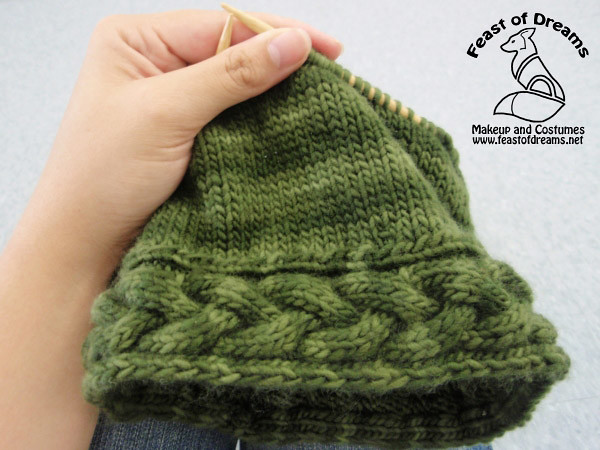Set against a light gray background, this color photograph in landscape orientation captures a hand in mid-motion, holding a dark green knit cap adorned with a chain design woven around its bottom edge. The right hand, belonging to a Caucasian individual, extends from the bottom left corner to the top left edge of the image. The thumb and forefinger of the hand delicately grasp the cap’s top, where two knitting needles, wrapped with green threads, protrude from the work in progress. The cap, displaying various shades of green, dominates the center of the image with its intricate weaves and patterns. In the upper right corner, a logo depicting a fox in profile is framed by the text "Feast of Dreams" above and "Makeup and Costumes" along with "www.feastofdreams.net" below, rendered in black line art. The realism of the handcrafted item and the photographic representation highlight the detailed craftsmanship involved.